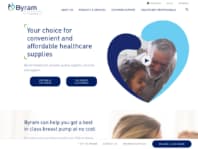This is a cropped screenshot depicting what appears to be the front page of a website. In the top left corner, the word "Byram" is displayed along with a logo. The screenshot is significantly blurry, making many details hard to discern. However, across the top header, four categories are faintly visible. 

Prominently featured in the body of the page, near the top left, is a large blue-font slogan that reads, "Your choice for convenient and affordable health care supplies." To the right of this slogan is a dual-colored heart icon, with a darker blue on the left and a lighter blue on the right. Centrally located is an interactive media element – a photo of a man and a young child with a triangular play button overlay, indicating a video player.

Towards the bottom, there's additional blue text; on the left side, the text is slightly smaller. Visible just below this text is the top of a woman's head, adjacent to a thumbnail image on the right. Dominating the bottom-right corner is a large blue button. The entire webpage remains notably blurred and reduced in size, reflecting the overall low clarity of the screenshot.